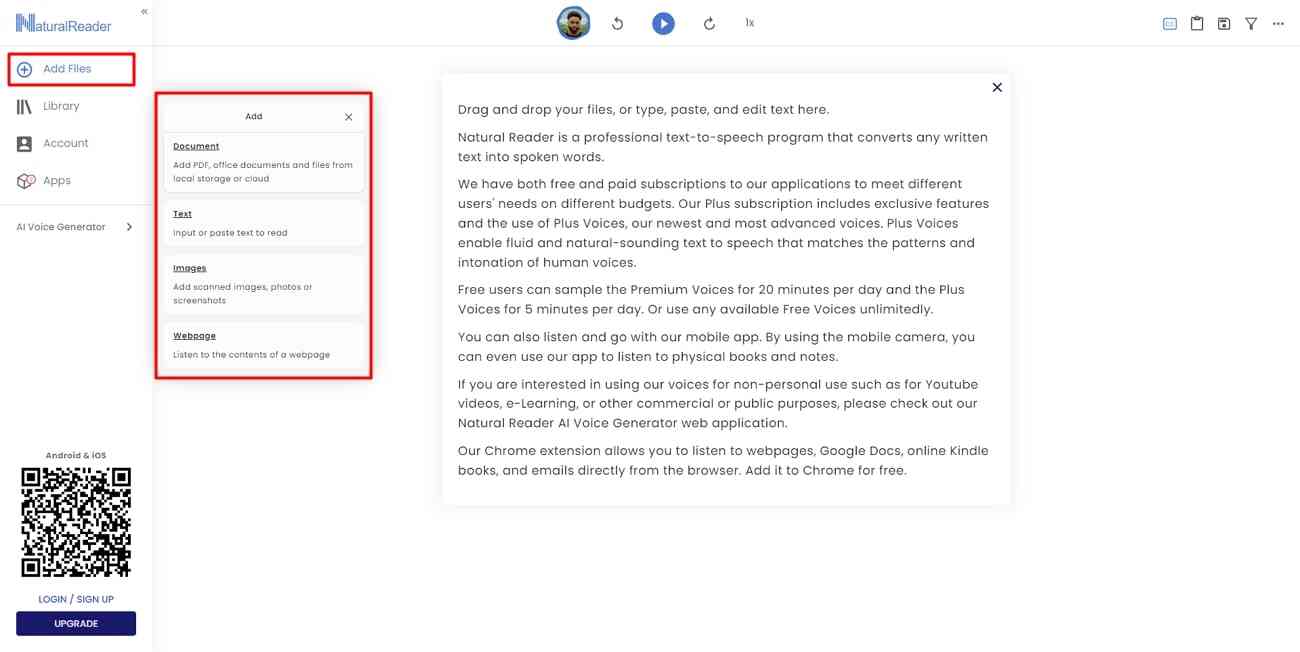This image is a cropped screenshot of the Natural Reader software interface. On the left side, there's a narrow vertical panel featuring the Natural Reader logo in blue at the top. Below the logo is a vertical list of options, with the option "Add Files" prominently highlighted within a red box. 

To the right, a pop-up box has expanded, triggered by selecting "Add Files." The pop-up is titled "Add" and offers four choices: Document, Text, Images, and Webpage, all encapsulated within a red border for emphasis. 

In the center of the interface is a large instructional white box with an 'X' at the top right corner for closing the box. The box provides guidance to users, stating, "Drag and drop your files or type, paste, and edit here." 

Natural Reader is described as a professional text-to-speech program that transforms any written text into spoken words. This description continues in three additional paragraphs beneath the instructional text.

At the bottom left of the screen is a sizable QR code. Directly below the QR code, the options "Log In" and "Sign Up" are presented in blue text. Further below, a prominent button labeled "Upgrade" is visible.